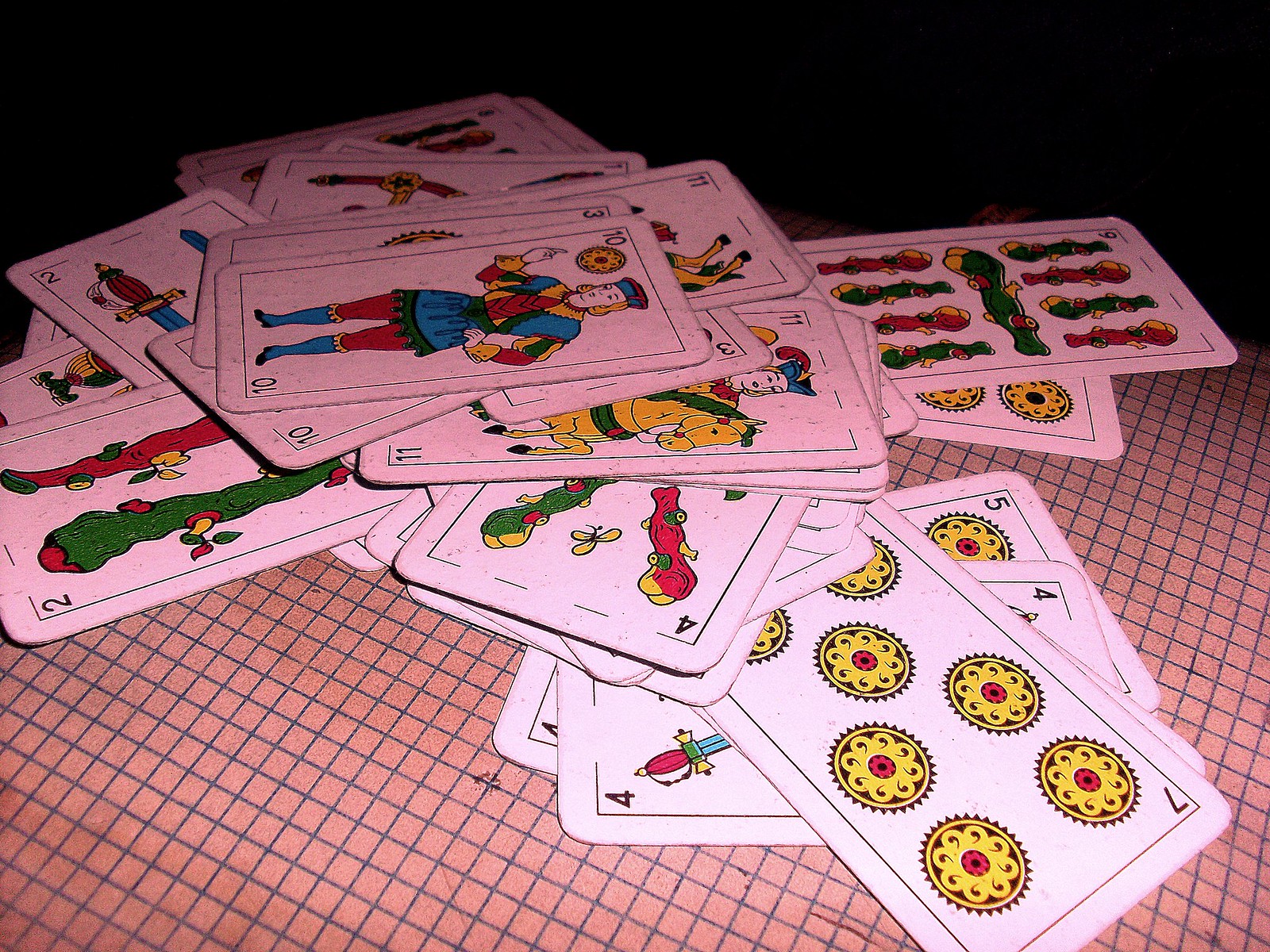The photograph features a plethora of playing cards arranged on a surface that resembles graphing paper, characterized by a grid of gray squares set against a reddish background, likely a fabric. The cards, totaling around 20 to 30, exhibit an antiquated design reminiscent of tarot cards, suggestive of Spanish playing cards. Among the suits displayed, one can identify coins, clubs, and swords, which are traditional elements of the Spanish deck.

The designs are intricate and varied. One card, a seven, showcases black circles adorned with a yellow spiral pattern and a red dot at its center. The clubs are depicted in an array of colors, including green and red, each embellished with yellow accents and small leaves sprouting from them. The topmost card in the arrangement is a ten of jacks, featuring a jack with yellow blonde hair and a colorful outfit dominated by shades of blue and green. His attire includes red tights and blue boots, and he is depicted pointing upwards. Another suit, the swords, is represented with a brown handle and a bluish blade, adding to the detailed and vibrant imagery of the collection.